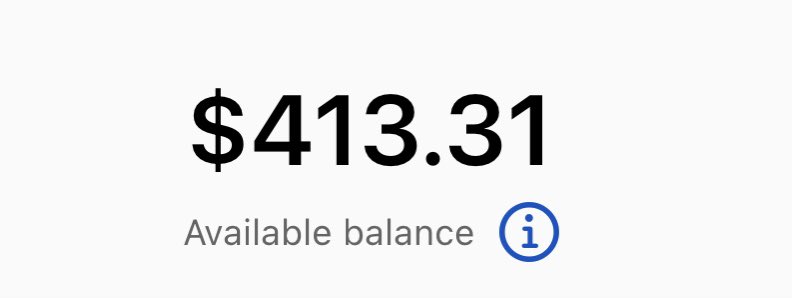The image features a light gray rectangular box. Prominently displayed in large, bold black font in the center of the box is the amount "$413.31". Directly beneath this figure, in smaller gray text, the phrase "Available Balance" provides additional context. To the right of the amount, there is a blue-bordered circle enclosing a lowercase "i," indicating an informational icon. The remainder of the box is unoccupied, presenting a clean and minimalist design with ample empty space.